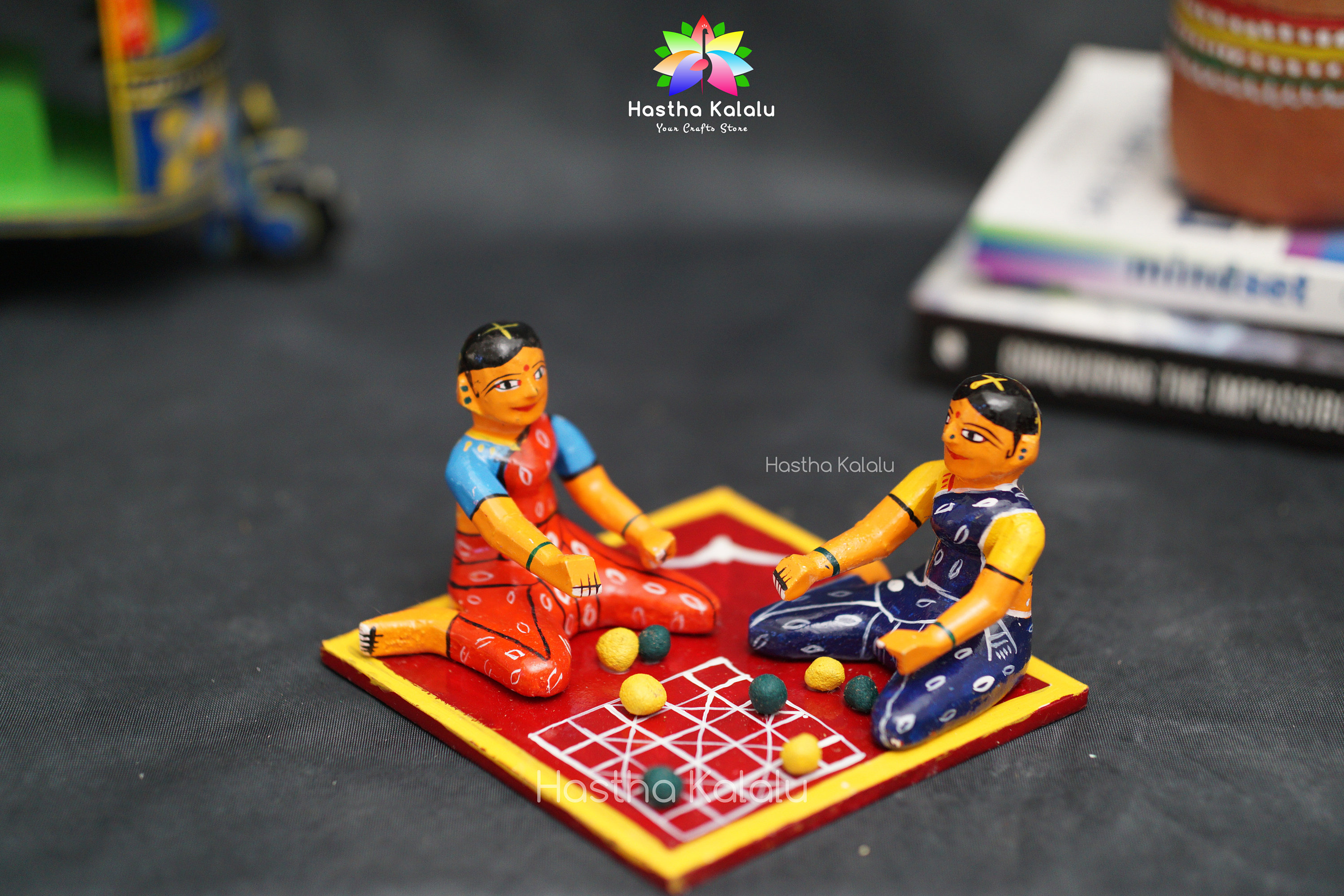The image depicts a detailed clay sculpture of two Indian figures engaged in a game. A logo reading "Haspa Kalulu" (or possibly "Hasta Ka Lalu") sits prominently at the top center of the photograph. The background features a blurred assortment of books and colorful objects, with a brown cylinder also visible. The figures, made with intricate pottery craftsmanship, sit on a black floor and place a red and yellow mat with a white crisscross grid design. Yellow and green balls are scattered around, some positioned on the mat's grid and others in their laps. Both figures have black hair adorned with a gold 'X' and wear green earrings. They have a distinct Hindu appearance, with red dots between their eyebrows. The left figure is dressed in a blue shirt and red sari, while the right figure is in a blue dress. Their legs are folded behind them, and they have their fists outstretched as if they are actively engaged in playing the game.